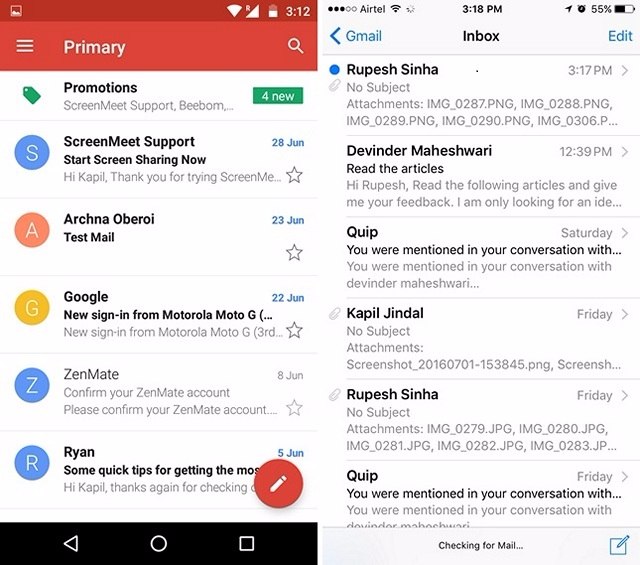This image shows two mobile screenshots of Gmail inboxes displayed side by side. The screenshot on the left features a red bar at the top and indicates it was captured at 3:12 PM. The inbox is in the "Primary" tab, with a label for "Promotions" below it. There are four new promotional emails visible. The first email is from "Screen Meet Support" with the subject "Start Screen Sharing Now" dated 28 June, beginning with "Hi Kapil, thank you for trying Screen Meet...". The second email is from Archana Oberoi, titled "Test Mail." The subsequent emails include "Google: New Signup for Motorola Moto G," "Zenmate: Confirm Your Zenmate Account," and an email from Ryan titled "Some Quick Tips for Getting the Most" starting with "Hi Kapil, thanks again for checking in."

The screenshot on the right has a gray bar at the top. The top email is from Rupesh Sinha, which has no subject and contains multiple PNG attachments. Below this email, one from Devinder Maheshwari with the subject "Read the Articles" starts with "Hi Rupesh, read the following articles and give me your feedback." Another email mentions a conversation with Devinder Maheshwari from Kapil Jindal, also without a subject, containing several attachments and screenshots. Additionally, there is another email from Rupesh Sinha with various attachments, followed by an email from Quip.